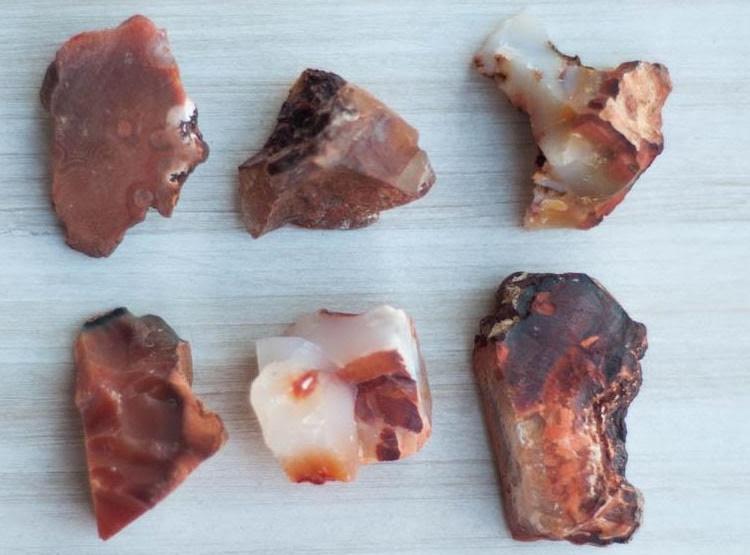This photograph, taken from above, displays six distinct rock specimens arranged on a smooth, gray board. The rocks are organized into two rows of three, with each rock roughly the same size but differing in shape and color patterns. The specimens predominantly feature a brown surface with irregular sides, adorned with white veining. 

On the top row, the leftmost rock is a dark reddish-brown with slight black and white discolorations. The middle rock has a black side, while the rightmost one is lighter with an area hollowed out and significant white presence. On the bottom row, the left rock, sharply angular like an arrowhead pointing down, is mainly dark brown with some black shading. The middle rock has the most white, resembling quartz with hints of brown, and is nearly cube-shaped. The rightmost specimen is oblong and the darkest of the set, with extensive dark areas and a nearly black top.

These rocks or mineral-based items, potentially mistaken for pieces of meat due to their pinkish hues with white elements suggestive of fat, exhibit intriguing forms and fascinating textures.